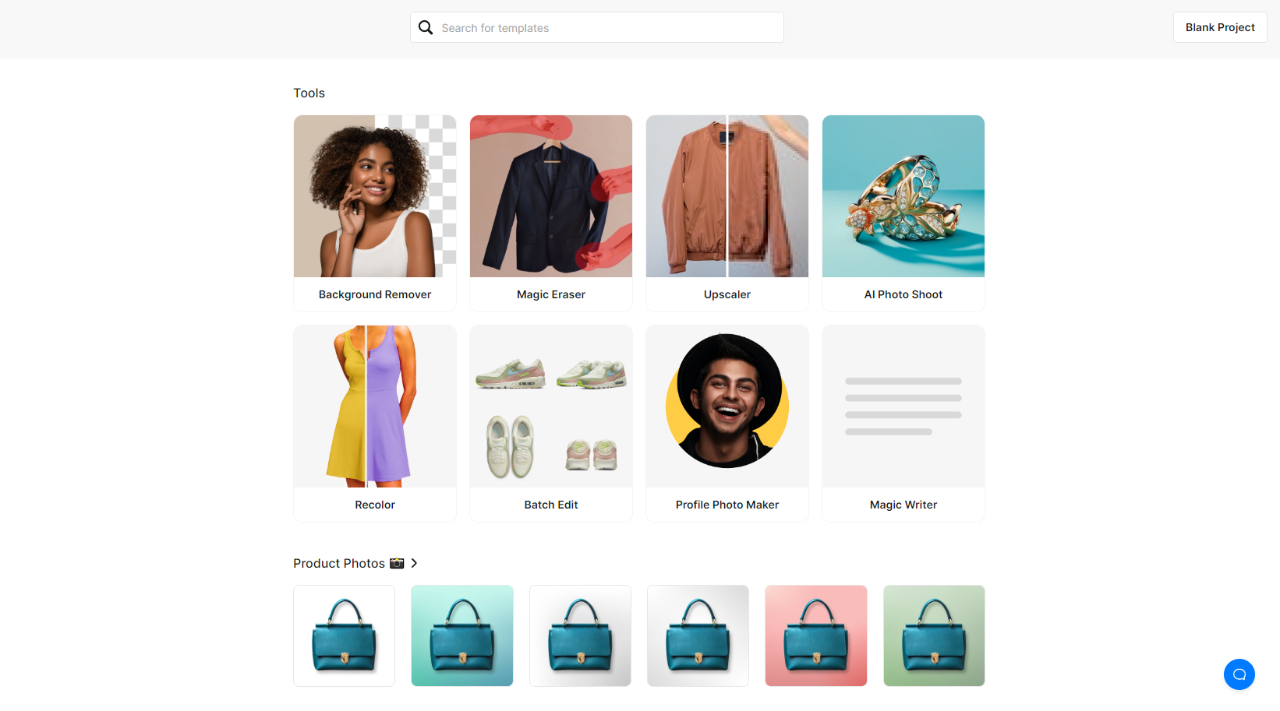This is a screenshot from an unidentified website. At the top of the page, there is a search bar featuring a black magnifying glass icon on the left, with the placeholder text "Search for templates" inside the bar. Below the search bar, the heading "Tools" is displayed.

The first image features an African American woman smiling and looking to the right, with her wavy, short dark hair framing her face. Her right hand is gently touching her right cheek. Below her image, the caption reads "Background Remover."

The next image shows a black blazer hanging on a wooden coat hanger, marred by visible red smears. The caption beneath this image is "Magic Eraser."

Following that, there is an image of a brown sweater. The left half of the image is clear while the right half is blurry, indicating a focus effect. The caption underneath reads "Upscaler."

Next, two jeweled rings are showcased against a turquoise surface and background. This image is labeled "AI Photo Shoot."

In the subsequent row, a photograph depicts a tank dress split into two colors: yellow on the left side and purple on the right. The caption below this image is "Recolor."

The following image displays various sneakers: a single sneaker and a pair of sneakers on the top row, and on the bottom row, a pair of sneakers viewed from above and from the back. The caption below reads "Batch Edit."

Then, a photograph of a young man smiling directly at the camera is presented. He has tan skin and is wearing a black hat. The caption for this picture is "Profile Photo Maker."

Next to the man's photograph, there is a gray square containing four horizontal gray lines. Below this square, the caption reads "Magic Writer."

Finally, an area labeled "Product Photos" showcases six images of the same turquoise-colored purse, each set against different colored backgrounds. The backgrounds, from left to right, are white, turquoise, white, white, pink, and green.